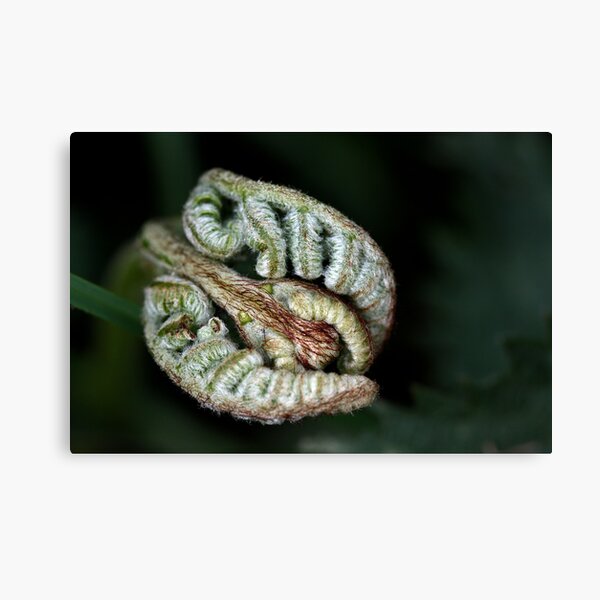The image features a photograph of a soon-to-blossom fern leaf prominently situated slightly to the left of the center against a light gray backdrop. The background of the image is blurred with green hues, suggesting a forest or woodland setting. The fern leaf itself is in early stages of growth, with its leaves still curled up and framed by white, cotton-like strands that add a delicate texture to the composition. Red streaks resembling veins run through the fern’s main stem, which branches out into four segments—two central ones and two larger outer ones. The colors present in the image include light gray, black, green, red, maroon, and light blue, enhancing the budding fern's intricate details. The photo appears to be presented in a circular frame, akin to a slide in a presentation, emphasizing the central focus on the developing fern leaf.